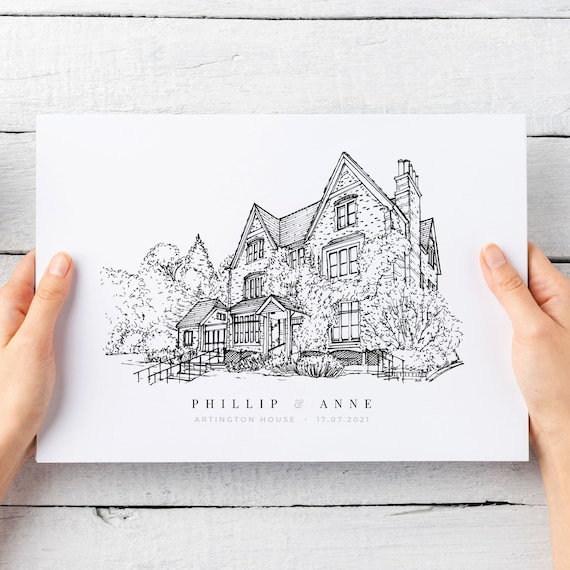In this image, a pair of Caucasian female hands firmly hold a stiff white paper, perhaps a poster board, featuring a detailed black-and-white ink sketch of a stately home. The sketch vividly portrays the exterior of the Philip and Ann Ardington House, dated 17-07-2021. This house, characterized by its stone (or possibly brick) facade, includes notable architectural elements such as a chimney on the right, two prominent front peaks, and a centrally located entrance with a covered porch to the left, accessible via stairs. Surrounding the house are lush trees and shrubs, enhancing its grandeur. The backdrop against which the paper is held consists of weathered, white-painted wooden planks, which might be part of a fence or table, adding a rustic touch to the scene.